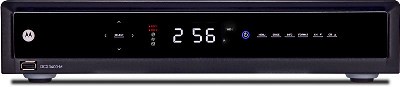The image features a black clock radio set against a white background. The clock radio has a sleek design with a small white circular emblem on one end that resembles the letter 'M'. The face of the clock radio is accented with a silver trim, and it displays the time as 2:56. Various buttons adorn the surface, catering to different functions like setting the time and selecting stations. It rests on two light gray, rounded feet that provide stability. Additionally, there is a small rotary dial for tuning to different AM and FM stations. The overall compact and sophisticated design makes it a pleasant and functional addition to any room.